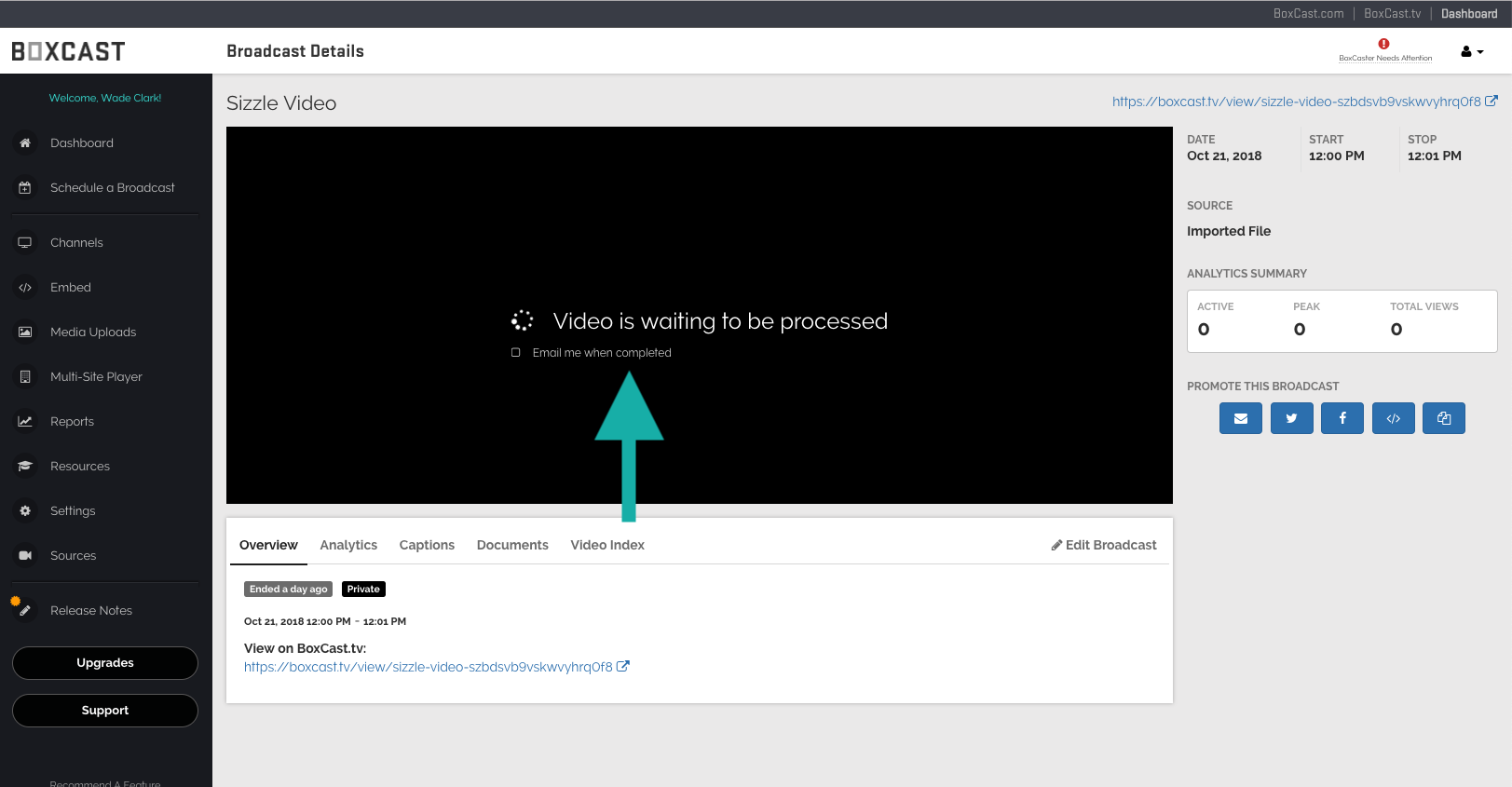The image depicts a desktop website interface designed for video management and playback. The user interface features a black left navigation bar adorned with white text and icons. At the top of this navigation bar, a friendly "Welcome Wade Clark" message is prominently displayed. The Nav bar includes various options such as Dashboard, Schedule a Broadcast, Channels, Embed, Media Uploads, Multi-site Player, Reports, Resources, Settings, Sources, and Release Notes. Below these options, there are two oval buttons with black backgrounds, gray outlines, and white text—one named "Upgrades" and the other "Support."

Central to the page, a header labeled "Sizzle Video" sits above a large black rectangle designed to preview videos. Currently, this section indicates that the "video is waiting to be processed," with a blue arrow pointing toward this text. Beneath it is a checkbox offering to "email me when completed."

Below the video section, a white box contains several tabs: Overview, Analytics, Captions, Documents, and Video Index. There is also a link to the video being uploaded.

On the right-hand side, there are fields displaying important details such as the URL to the video, the date, start and stop times, source information, an analytic summary, along with options to promote the broadcast via multiple social media channels.